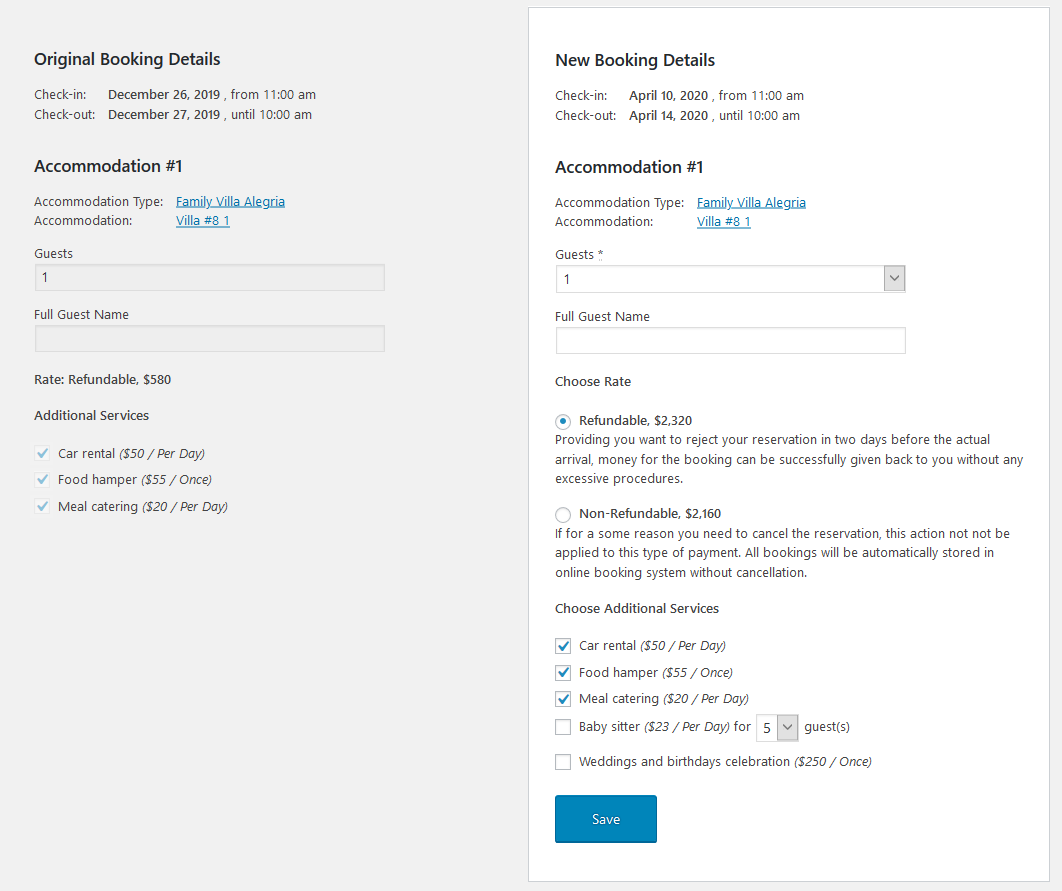The image features a split-page design reminiscent of an open book. The left side of the image has a grayish background, while the right side is white. This layout starkly contrasts as it presents two halves of a booking form, detailing original booking information on the gray side and new booking details on the white side.

On the left gray page, the header reads "Original Booking Details." It outlines the reservation specifics:
- **Check-in Time**: December 26, 2019, from 11 a.m.
- **Check-out Time**: December 27, 2019, until 10 a.m.
- **Accommodation Section**:
  - Type: Family Villa
  - Location: Algeria
  - Villa Number: 8.1 (or 8-1)
- **Guests**: Lists one full guest, though the name remains empty.
- **Rate**: Refundable, $580
- **Additional Services**: Car rental, food hamper, and meal catering.

On the right white page, the header reads "New Booking Details." It updates the reservation with:
- **Check-in Time**: April 10, 2020, from 11 a.m.
- **Check-out Time**: April 14, 2020, until 10 a.m.
- **Accommodation Section**:
  - Type: Family Villa
  - Location: Algeria
  - Villa Number: 8
- **Guests**: One guest
- **Rate**: 
  - Refundable: $2,320 (bubbled in)
  - Non-refundable: $2,160
- **Additional Services**: Chosen services include car rental, food hamper, meal catering, with additional options for babysitter and weddings listed but not selected.